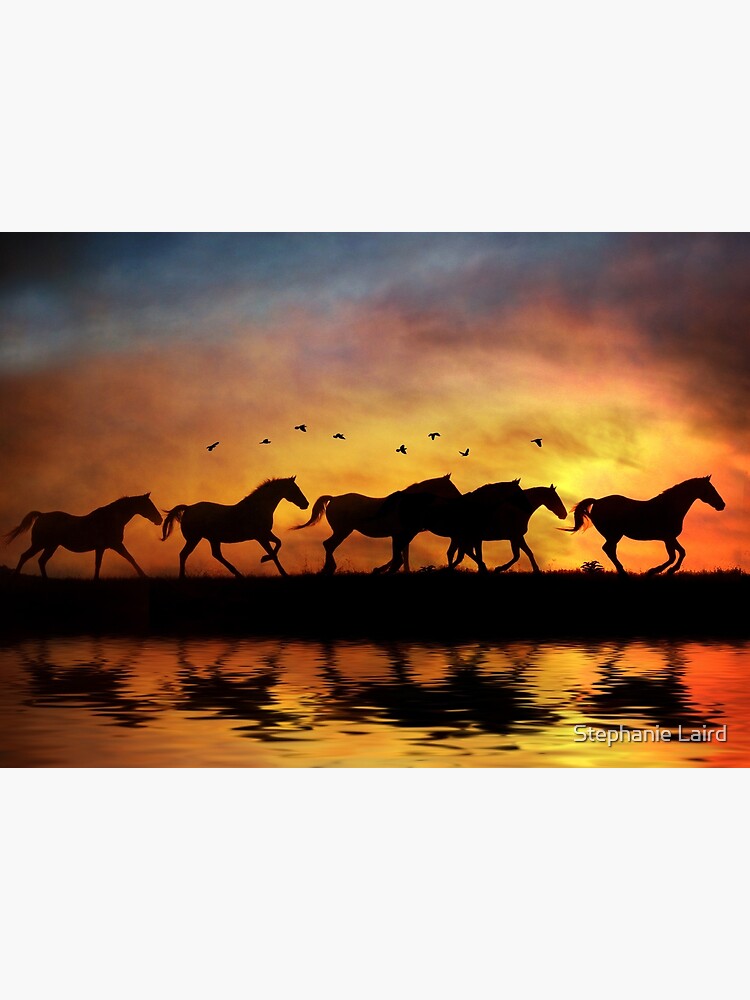This highly detailed and stylistic photograph, likely taken by Stephen L.A. Laird, captures a striking scene at either sunrise or sunset. The top of the sky transitions from dark blue to a gradient of orange and yellow hues, with an overlay of clouds. In this evocative setting, six dark-colored horses are seen running from left to right. Beneath them, their silhouettes are mirrored in the body of water they run beside, enhanced by the glistening waves reflecting the orange glow of the sky. Above, seven or eight birds fly gracefully, adding to the dynamic composition of the image. The horses and their reflections dominate the foreground, creating a sense of movement and energy against the serene, yet dramatic backdrop.